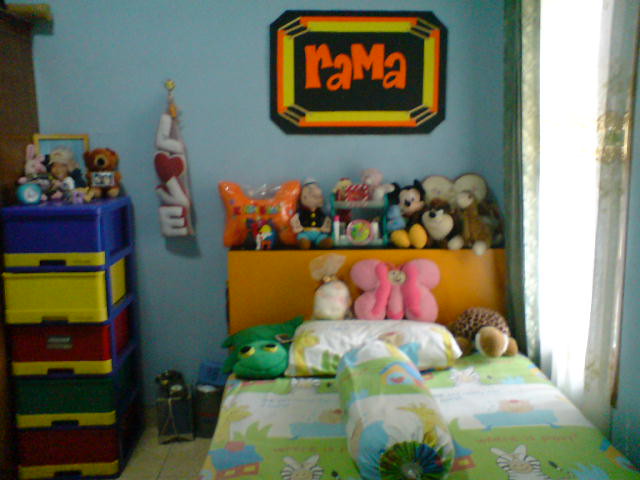The image depicts a cozy child's bedroom with walls painted a light powder blue. In the upper right-hand corner, a vibrant sign featuring the letters "R-A-M-A" in orange is displayed against a black background bordered by yellow, presumably indicating the child's name. Beneath this sign and bright window with curtains stands a child's bed adorned with a light green and white bedspread. The bed is filled with a delightful assortment of stuffed animals, including a green frog, a pink butterfly, a green snake, a brown turtle, and a small white stuffed animal, scattered across the bed and its headboard. To the left of the bed, a multi-colored chest of drawers in blue, yellow, red, and green is placed, topped with additional stuffed animals, enhancing the whimsical charm of the room.